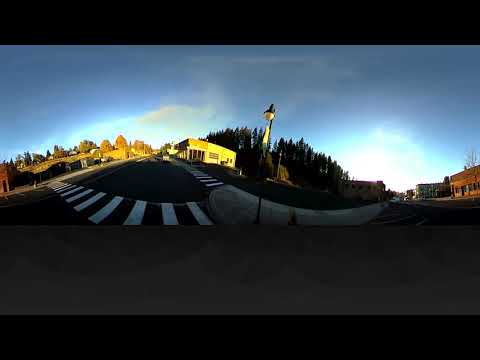This outdoor photograph showcases a transitional scene between residential and commercial areas, set against a backdrop of a blue sky that gradually lightens towards the horizon. Centrally featured is a black gravel-paved roadway that leads towards the camera, characterized by an apex curve to the right, and a white-striped crosswalk extending from the middle to the left side of the street. The visible light sources, with pronounced white sections, indicate it is late in the afternoon or nearing dusk, casting long shadows.

On the left, the landscape includes gently undulating hills adorned with a juxtaposition of tall dark trees and dense clusters of smaller trees extending to the horizon. Nestled into this wooded area is a small yellowish building accompanied by a light post. In the foreground, the vicinity contains the predominantly residential structures, homes set into the hillside, bathed in bright light yet contrasted by shadows in the foreground.

On the right side of the image, a distinct commercial area emerges where the road curves, featuring varied buildings that may serve as markets or shops. These structures differ visibly from the more uniform homes on the left. This side is also marked by a cemented sidewalk and further defined by a black structure extending horizontally across the backdrop, adding a prominent, linear element to the composition. The comprehensive description captures the intricate interplay of light, shadow, and the diverse architectural landscape, providing a vivid portrayal of the scene.